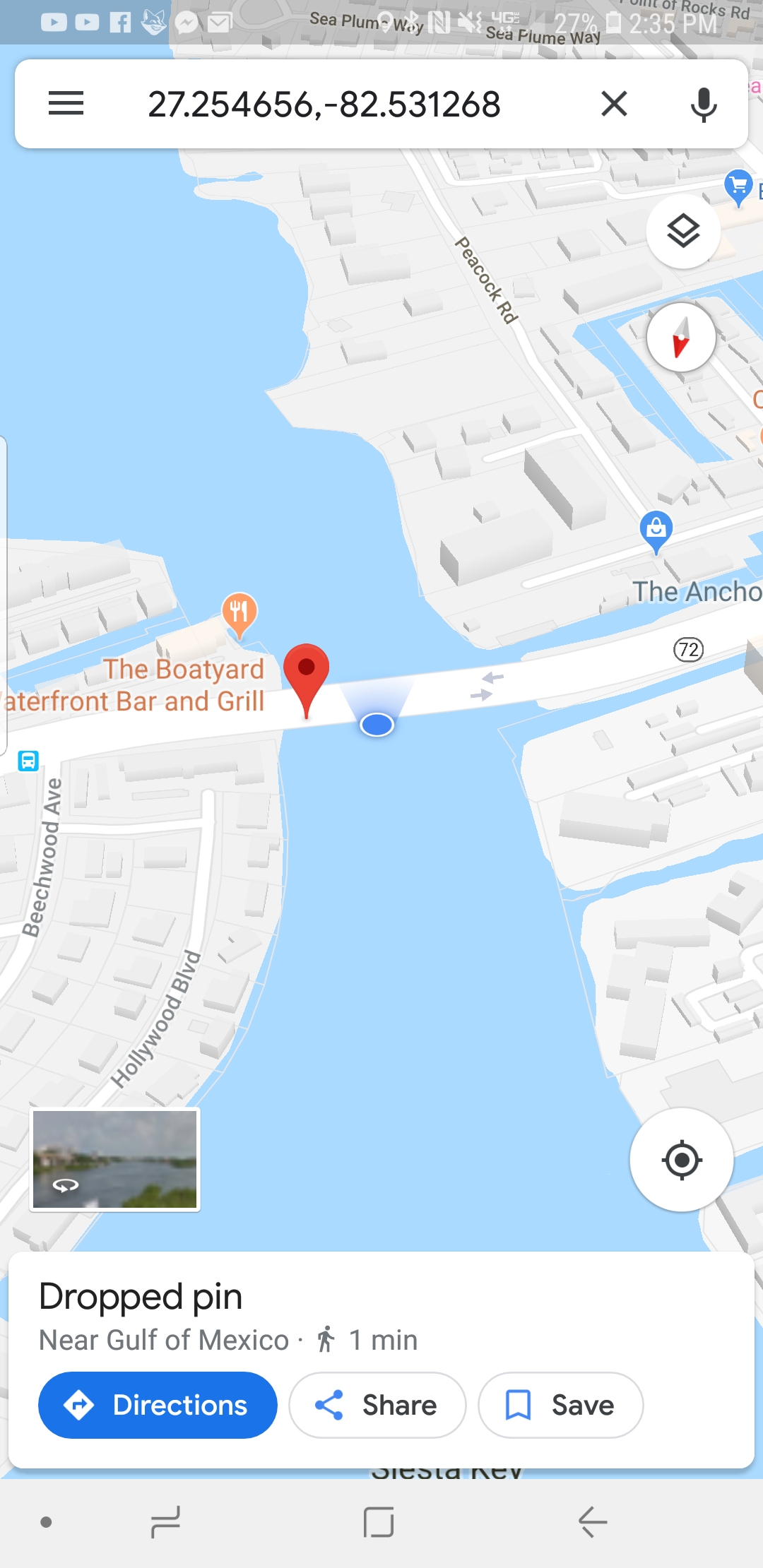The screenshot captures a phone screen displaying a map. At the top of the screen, the status bar shows various icons including YouTube, Facebook, and Messenger on the left, and a GPS icon, 4G signal strength, a 27% battery indicator, and the time, 2:35 PM, on the right. Just below the status bar, there is a search bar containing coordinates "27.25, -82.53" with an "X" button to clear the search and a microphone icon for voice input. The main portion of the screen features a map displaying an area with two landmasses separated by a large river or body of water. A bridge connects the two landmasses, and a pin is placed at the midpoint of the bridge.